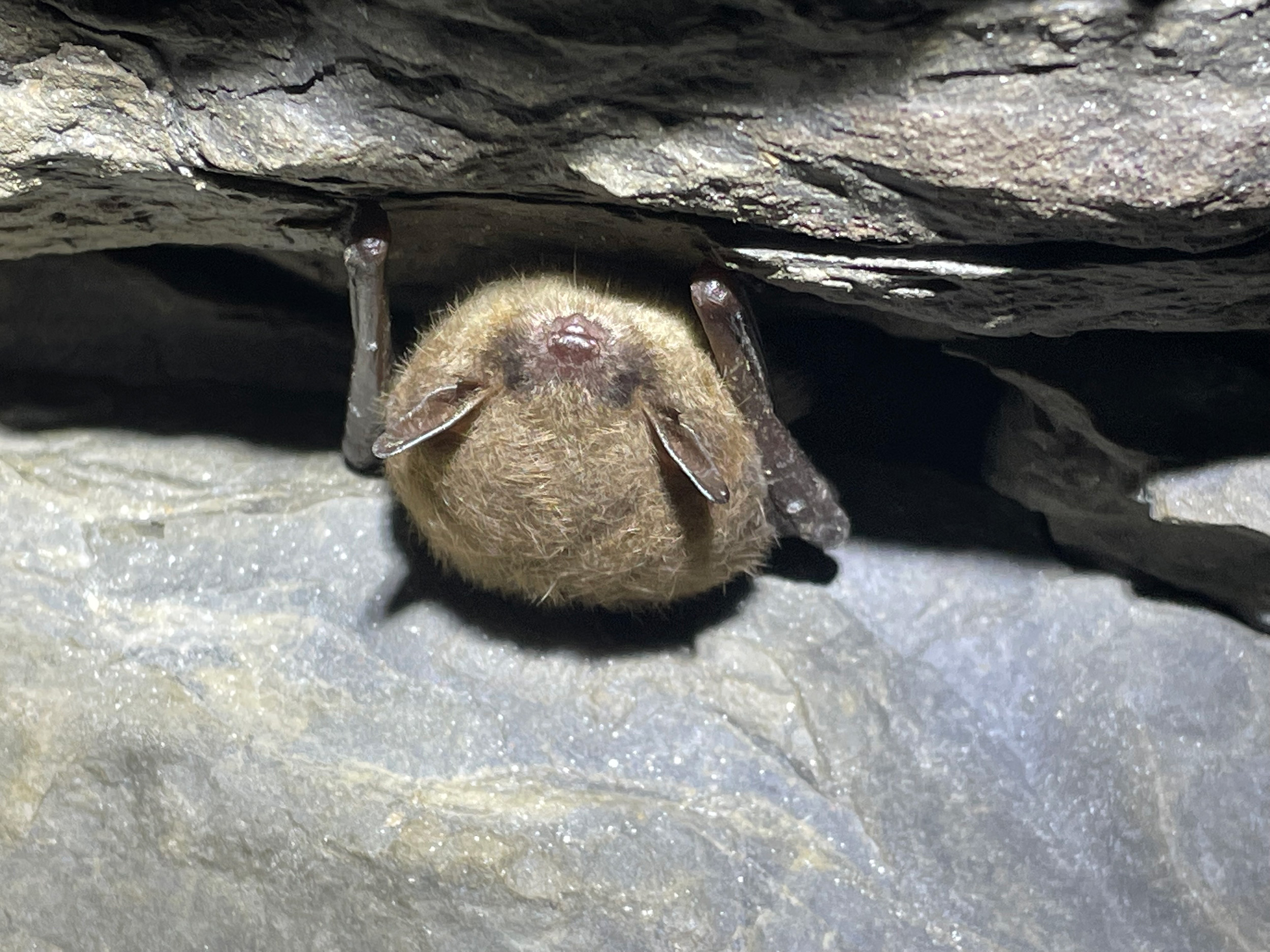The image depicts an upside-down bat nestled within a crevice of a large rock wall. The bat is suspended between two rocks—a beige, bluish-tinted rock on the bottom and a beige rock on the top. The bat's tiny ears are pointing downward, while its mouth and two front feet (or claws) are visible, touching the upper rock. The bat's back is covered in fine yellow fur, and its eyes are barely discernible as small slits beneath its ears. Sunlight illuminates the scene, casting shadows on the rocks and highlighting their jagged, shiny particles. The bat appears to be fast asleep, hanging securely within the crevice.